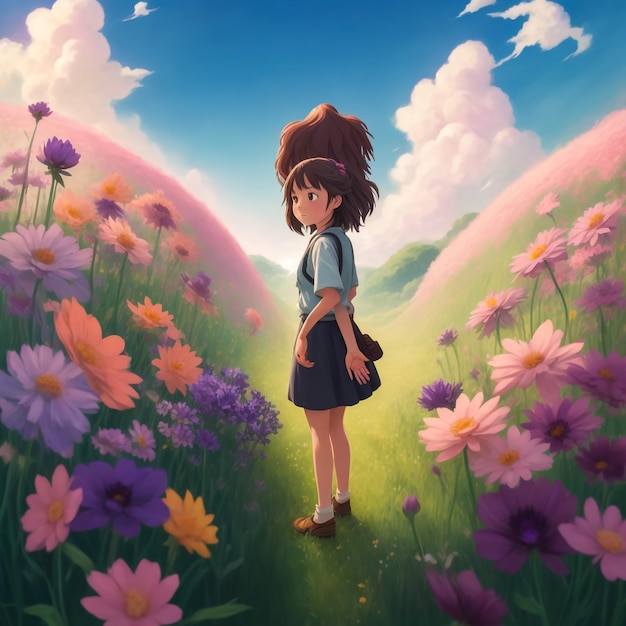In the image, there is a digitally rendered, AI-generated scene depicting a young girl with an unusual third arm emerging from her back. She stands amidst a picturesque field dominated by vibrant wildflowers in pink, purple, white, and yellow hues. The girl, with her dark brown, voluminous hair tied into a high puffy ponytail, wears a white and blue attire that resembles a uniform consisting of a white t-shirt with a blue and black sweater vest over it, a dark blue skirt, brown shoes, and white ankle socks.

The landscape surrounding her consists of rolling green hills, featuring a distinctive U-shaped dip in the middle. Atop these hills, pink flowers blend with the green, possibly reflecting the light or consisting of actual pink grass. A blue sky overhead is adorned with large, fluffy white clouds, adding to the serene atmosphere. The girl is positioned slightly to the left, facing forward but angled to the side, seemingly lost in thought within the natural beauty that surrounds her.